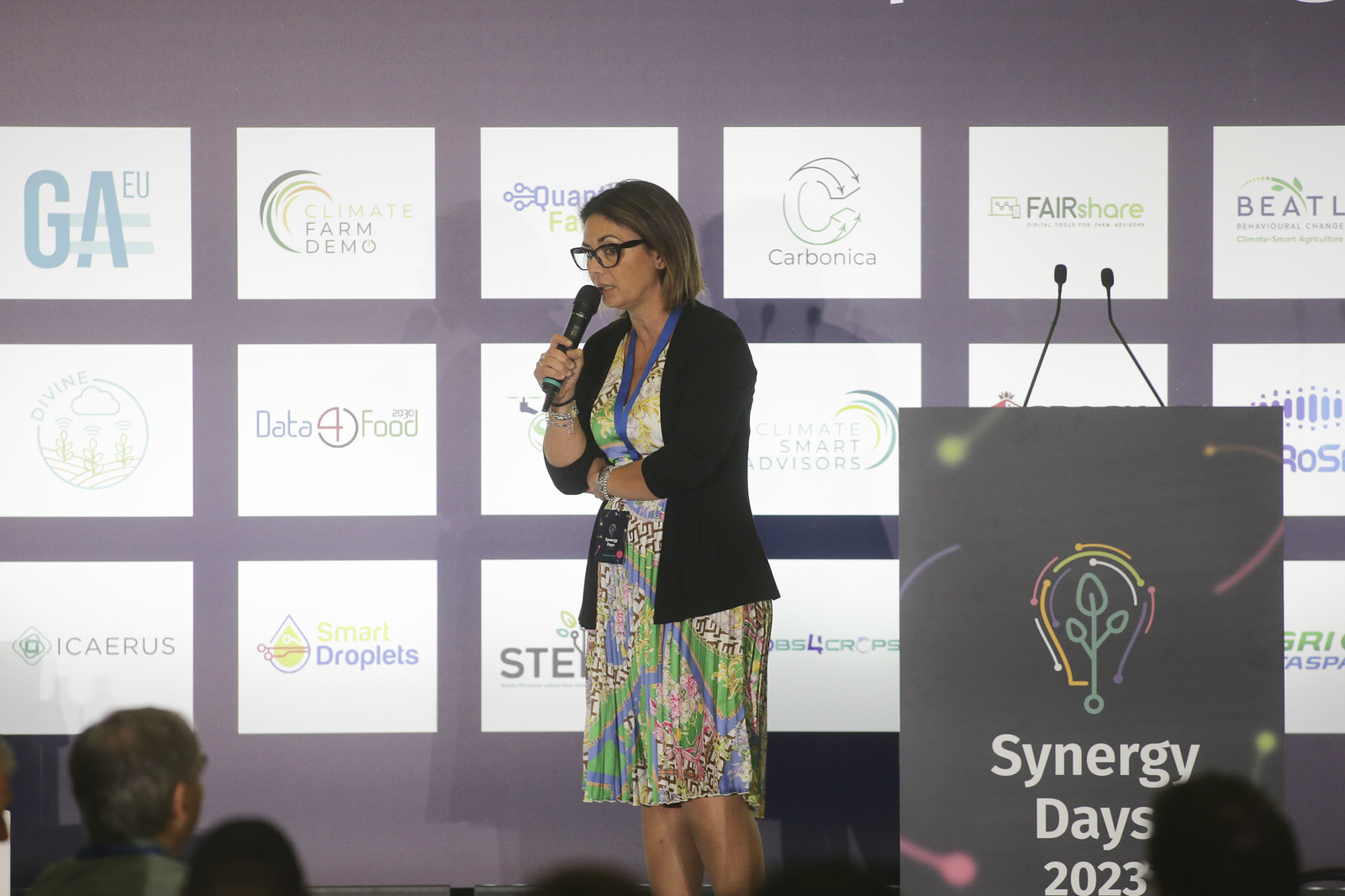In the photograph, a woman stands confidently on a stage, addressing an audience as she speaks into a handheld microphone. Positioned to the left of a sleek, black lectern, which prominently displays the words "Synergy Days 2023" alongside an emblem of a lightbulb entwined with leaves, she exudes a professional aura. The stage's backdrop is a modern, illuminated display consisting of numerous white squares, each housing logos of various corporate sponsors such as Climate Farm Demo, Carbonica, and Fair Share, among others. The background hue transitions from purple to gray, enhancing the contemporary feel of the setting. Wearing dark-rimmed glasses and a blue-lanyarded name tag, she is dressed in a vibrant, multicolored floral dress paired with a black cardigan. Her hairstyle, a short bob that neatly frames her face, complements her poised appearance as she engages with her audience, whose heads can be seen in the foreground of the image.